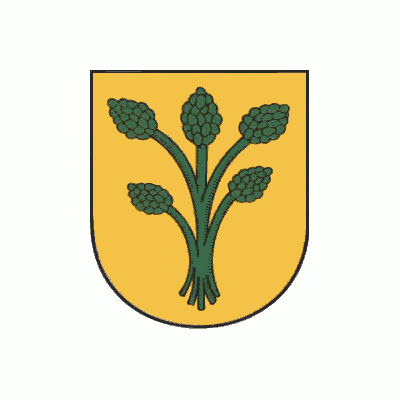The image is a crest or badge with a U-shaped outline that has a flat top and a curved bottom. The background is yellowish-orange, bordered by a thin black line. Central to the design is a depiction of five green asparagus stalks. These stalks originate from a single base and then split upward into individual stalks, with three straight up in the center and two smaller ones extending to the sides. Each asparagus stalk has a thin black border. The overall effect is a simple, clean design with no text, figures, or additional objects.